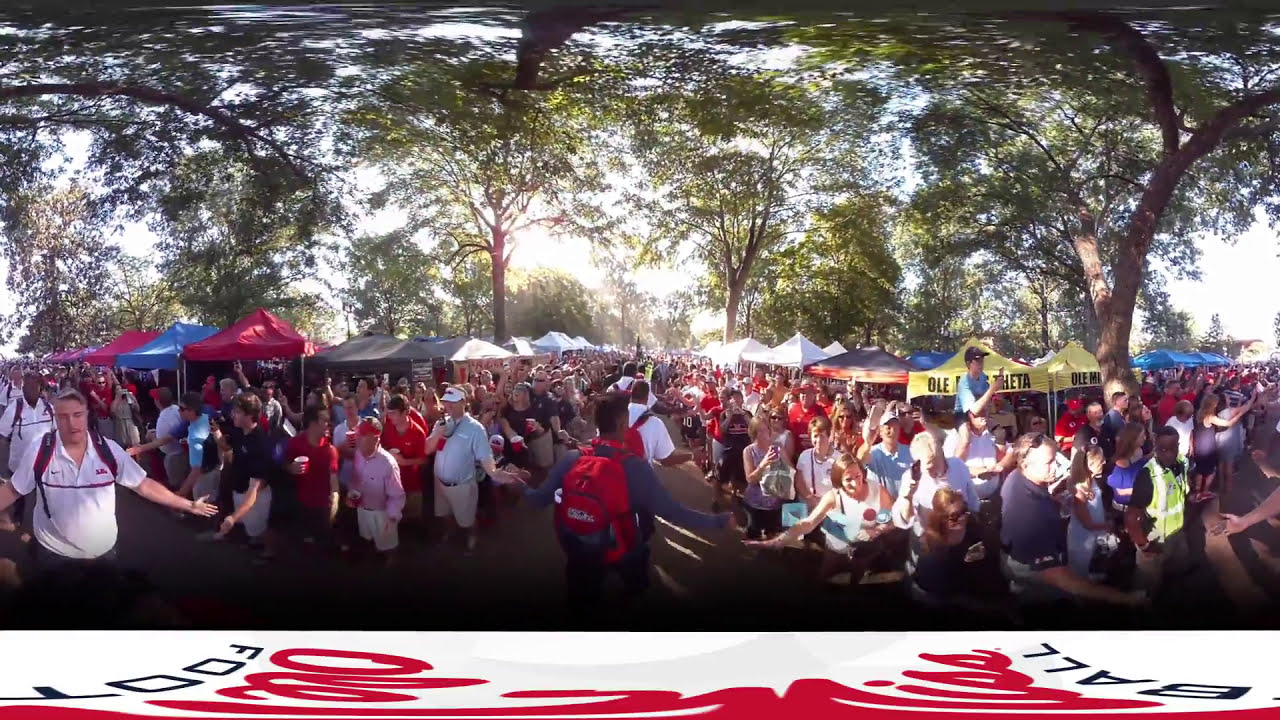The image captures a bustling outdoor fair or festival set under a mid-morning sun with a clear blue sky. Numerous awning structures in an array of colors—red, blue, white, gray, yellow—line a street, creating shaded areas where a large crowd gathers. Hundreds of people navigate through and beneath these canopies, contributing to the lively and crowded atmosphere. Tall trees with lush leaves surround the event, offering additional shade. Prominent individuals include a man in a white shirt with outstretched arms on the left, a man with a red backpack in the center, and a man wearing a greenish-yellow vest on the right. The overall scene is vibrant and dynamic, filled with the energy and movement of a densely packed crowd enjoying the fair.